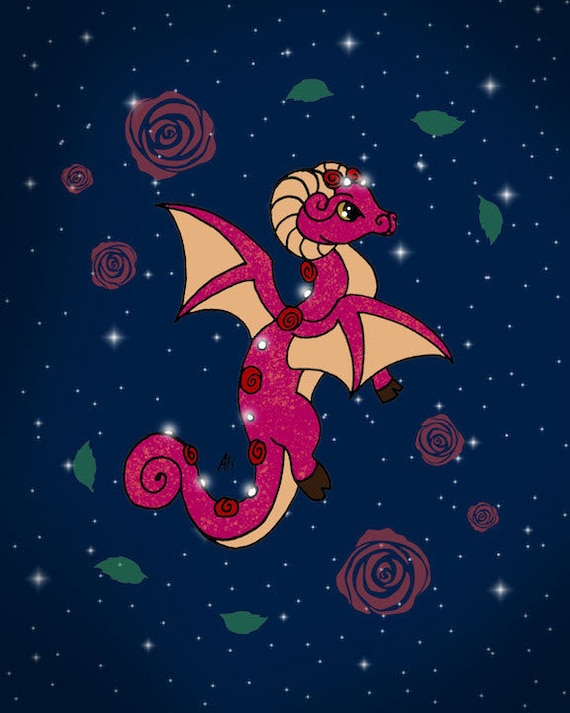This image showcases a detailed, cartoonish illustration reminiscent of the My Little Pony artwork style. The backdrop is a dark blue, resembling a night sky adorned with scattered white stars of varying brightness. Situated prominently in the center is a pink and peach-colored dragon with a feminine appearance. She is upright, stabilized by her coiled tail. Facing the right, the dragon has a distinctive curly horn-like structure behind her head, matching tan hooves, and tan highlights on her chest, belly, and wing edges. Her wings are prominently extended, displaying the tan underbelly that extends from her chest to the base of her tail. Adding to the enchanting scene are sporadically placed salmon-colored rosebuds and three floating green leaves located above the dragon's head on the right. The combination of these elements creates a whimsical, celestial-themed artwork that blends stars, roses, and a charming dragon into a cohesive and captivating visual.